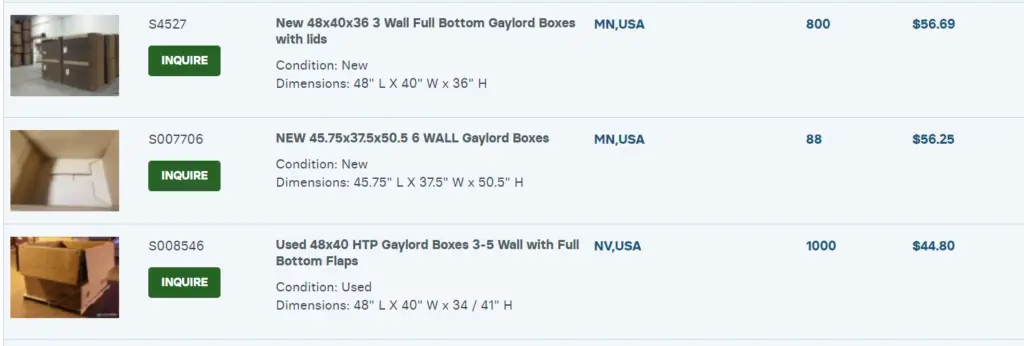This image depicts an online shopping website that appears to specialize in selling various types of boxes. The focus is on different box listings with their respective prices and specifications. 

1. **New 48" x 40" x 36" Three-Wall Full Bottom Gaylord Boxes** 
    - Price: $59.69
    - Quantity Available: 800

2. **New 45.75" x 37" x 50.56" Gaylord Boxes**
    - Country: USA
    - Price: $56.25
    - Quantity Available: 88

3. **Used 48" x 40" HTP Gaylord Boxes with Three-Wall Full Bottom Flaps**
    - Quantity Available: 1,000
    - Price: $44.99 each

The website provides detailed specifications, pricing, and availability for each type of box, helping potential buyers make informed decisions.